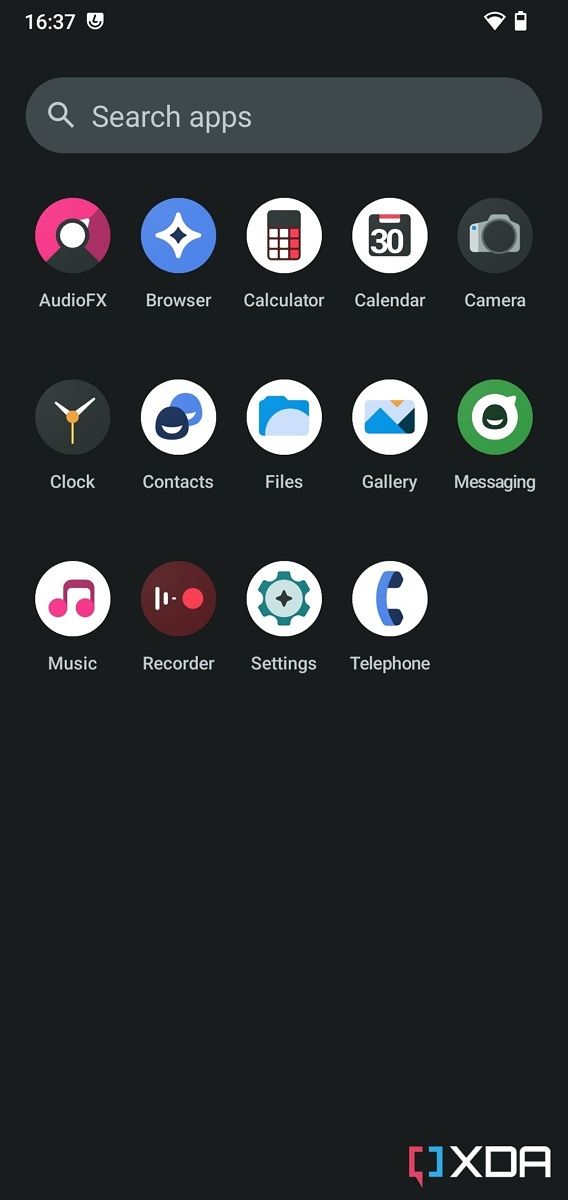The image shows a dark gray rectangular interface, presumably a device's screen. At the top, the time is displayed as "16:37". Next to the time, there is an icon resembling an upside-down shield with indecipherable black markings inside it. Additionally, there are icons for Wi-Fi signal and battery status.

Below the top bar, there's a light gray rectangular search bar with magnifying glass icon and the text "Search apps". This search bar is slightly bulged on both the left and right sides.

Underneath the search bar, there's a grid of app icons with corresponding labels: 
- Audio Effects: represented by a pink partial circle with a black section and a black outlined white circle in the middle.
- Browser: icon not described.
- Calculator: depicted as a calculator.
- Calendar: shown as a calendar.
- Camera: illustrated with a camera.
- Clock: icon not described.
- Contacts: icon not described.
- Files: icon not described.
- Gallery: icon not described.
- Messaging: icon not described.
- Music: icon not described.
- Recorder: icon not described.
- Settings: icon not described.
- Telephone: icon not described.

At the bottom of the screen, there is a logo consisting of a pink and blue shape, together resembling a capital "Q" but split apart with a dividing line; the left side is pink and the right is blue. Adjacent to this logo, "X DA" is written in white text.

Each app icon typically represents its function clearly, such as the calculator showing a calculator and the calendar showing a calendar, although some icons, like the one for Audio Effects, are more abstract and harder to interpret.